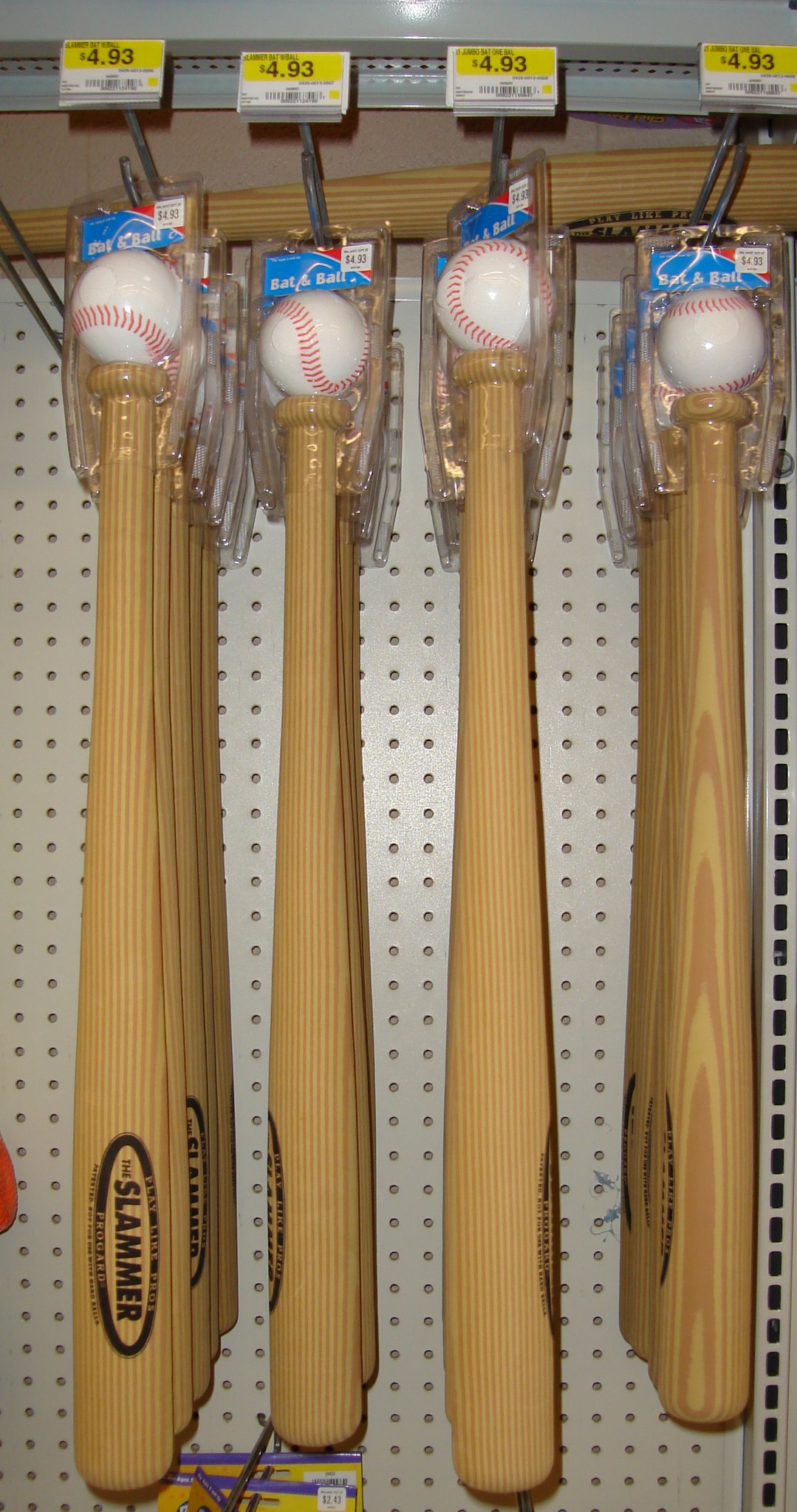The color photograph depicts a store display of baseball bat and ball sets. The bats, crafted from plain wood with visible grain, are branded with the name "Slammer" in a black oval on the widest part of the bat. Each set includes a traditional white baseball with red stitching, encased in a clear plastic clamshell attached to the handle of the bat to ensure the ball stays securely in place. The display is organized on a perforated off-white pegboard, with metal pegs holding up the bats. Price tags above each row indicate that each set costs $4.93. The neatly arranged rows feature bats in various sizes, all hanging from S-hooks, creating an orderly and inviting retail presentation.